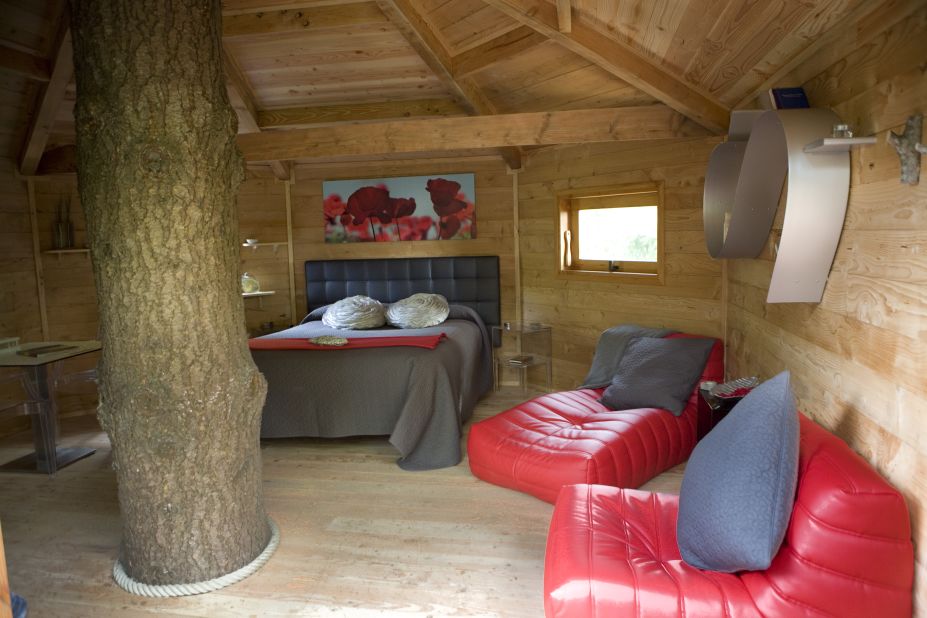The photo captures the interior of an exquisitely designed treehouse, resembling a luxurious resort more than a typical child's playhouse. Central to the room is a massive tree trunk, encircled by an expertly constructed wooden structure with walls, floors, and ceilings all meticulously crafted from tan-colored hardwood. The treehouse appears to be octagonal in shape, providing a unique architectural twist. A white rope at the base of the tree trunk ensures the space remains airtight.

The furnishings emphasize both comfort and style. A queen-size bed draped with gray blankets and accented by two decorative pillows stands against the back wall, suggesting a cozy place for relaxation. In the foreground are two distinctive red chairs that resemble a blend of bean bags and traditional seats, each adorned with a gray pillow. Additional seating includes a smaller red sofa-like chair positioned towards the bottom of the image.

A small wooden table on the left side complements the interior, and artwork, including an image of red roses above the bed, adorns the walls. There is also a unique sculpture that resembles a folded piece of metal, adding a touch of modern art to the rustic setting. A window on the center-right allows natural light to filter in, enhancing the warm and inviting ambiance of this exceptional treehouse retreat.